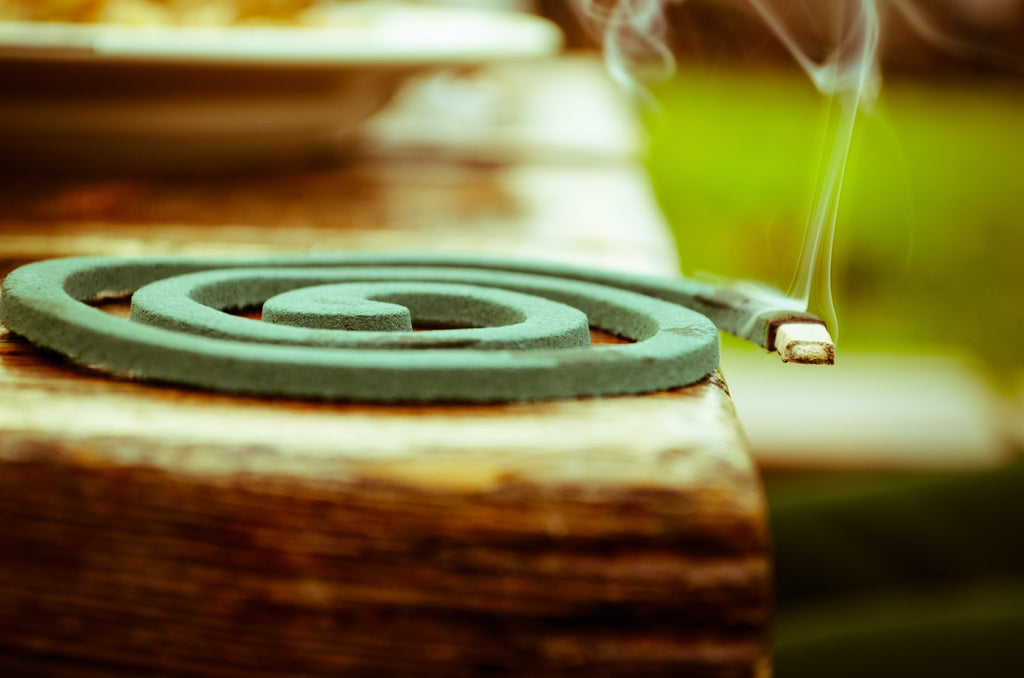This detailed color photograph, taken in landscape orientation, showcases an outdoor scene with a prominent mosquito coil lying flat on a medium brown wooden table surface. In the foreground, the medium green coil is centrally positioned, with its spirals neatly curling in on themselves. The end of the coil protrudes slightly over the edge of the table on the right and is visibly lit, glowing white with a wisp of thin white smoke rising from the burning end, exuding insecticide. The background of the image is blurred, revealing vibrant green colors on the right, suggestive of grass or foliage. To the left, a shallow flat white bowl with a wide rim rests on the table; though out of focus, it adds context to the setting. The photograph adheres to a photographic representational realism style, capturing an ordinary yet detailed moment of the mosquito coil in use.